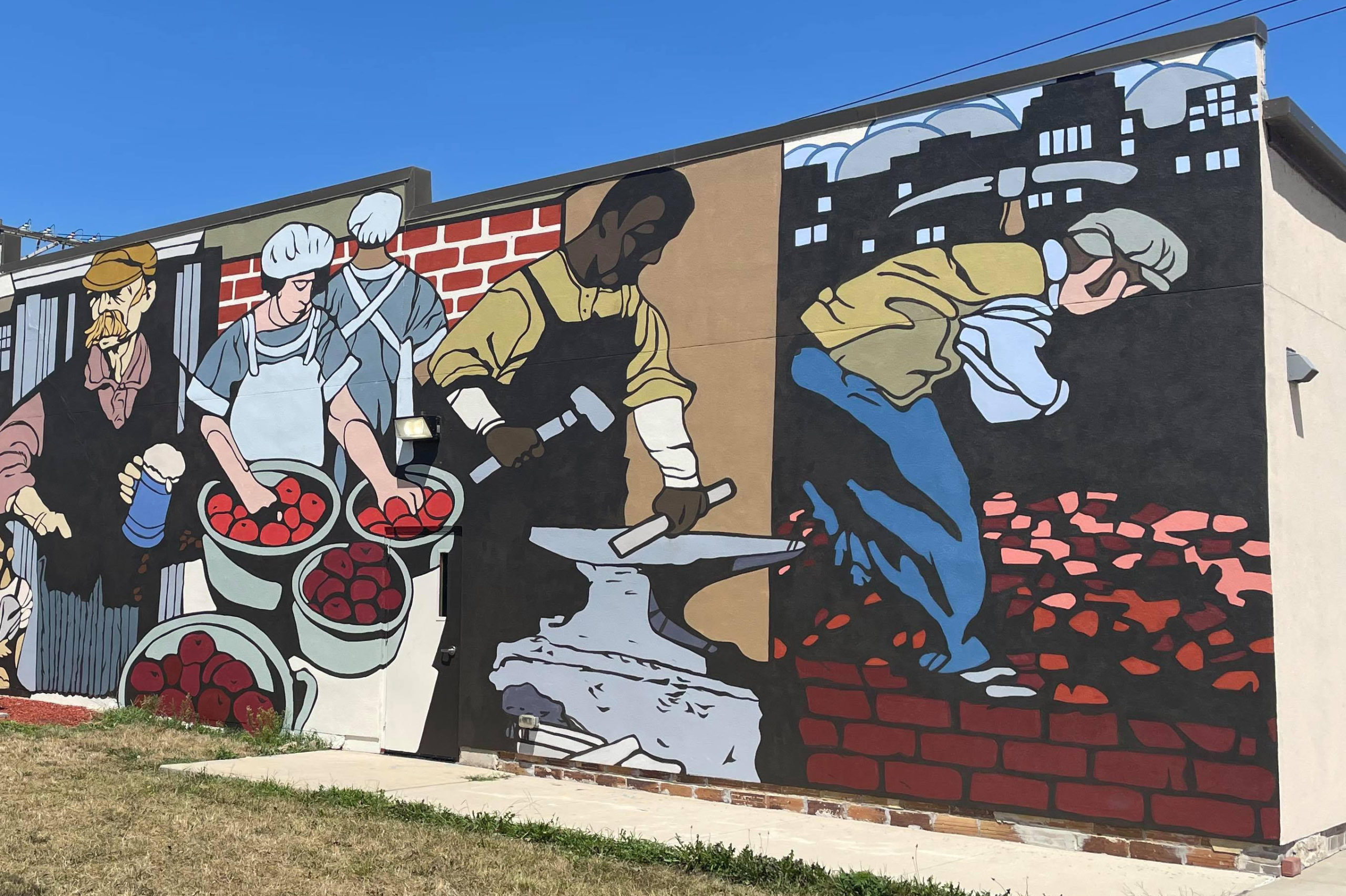In this landscape-oriented color photograph, we see a detailed mural painted on the exterior wall of a single-story building. The mural, rendered in a realistic and representational style, is situated along the backside of the building, which features a beige stucco facade and a red brick foundation. The scene is set outdoors with a clear blue sky and a well-maintained lawn bordered by a concrete sidewalk.

The mural itself is a vibrant and intricate depiction of various workers engaged in their respective tasks. Starting from the left, there is a man in a yellow hat and a pink shirt under a black vest, appearing to walk out of a doorway painted with red bricks. Next to him are two individuals in white cafeteria hats and aprons, handling red apples and metal buckets against a similar brick backdrop.

Towards the center, a dark-skinned blacksmith wearing a black apron and a yellow shirt hammers a piece of metal on a gray anvil, his focused expression captured in the lifelike detail of the painting. To his right, a man in a beige jacket, blue pants, and a gray cap bends over in a field of red and pink flowers, wielding a pickaxe over his chest.

Further to the right, a young boy in a yellow-brown shirt and a hat is depicted running over a pile of red bricks, while in the background, a black silhouette sits amidst blue smoke, adding a sense of depth and mystery to the artwork. The final figure on the far left holds a steinful of beer, gazing thoughtfully to the side.

This meticulously crafted mural could plausibly be a commissioned piece given its high-quality execution and the training evident in the artist's skill.